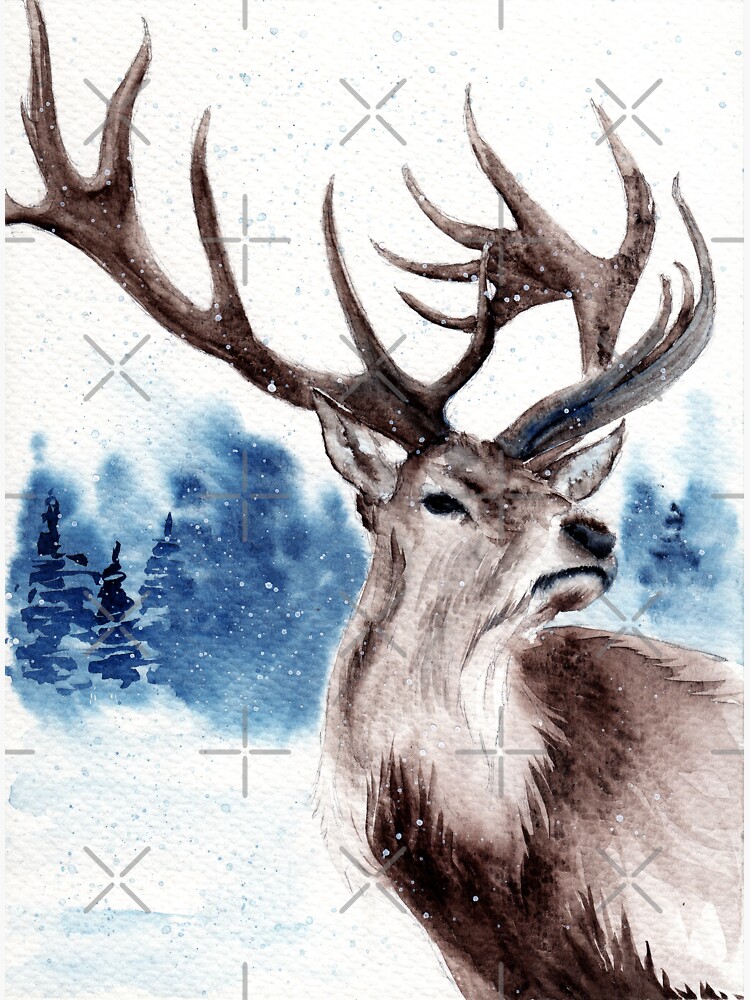This is a highly detailed color photograph of what appears to be a watercolor painting of a full-grown buck deer during wintertime. The backdrop is a snowy white landscape, dotted with dark blue and green fir and pine trees that create a cold, serene ambiance. The foreground features the majestic deer, with a colossal 20-point antler rack. His head is predominantly light brown, transitioning to white along his thick neck, and his body showcases earthy brown hues that blend naturally into the winter scene. The deer's large black nose and expressive eyes draw the eye, emphasized by the light brown fur on his head and chest. Snow is depicted with white splatters that add texture and realism to the scene, appearing both on the deer and the background. Over the entire image, there is a pattern of gray cross-hatch marks resembling a watermark, adding another layer of complexity to the artwork.